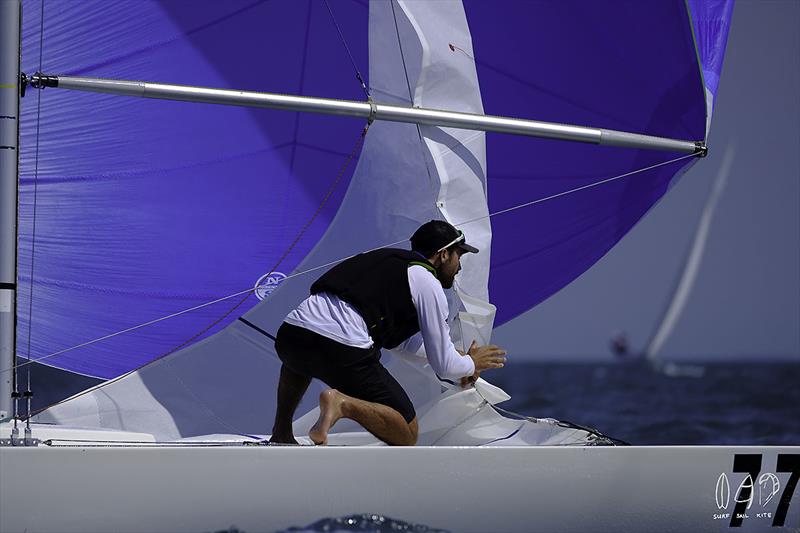The photograph captures a man actively working on a small, swiftly moving sailboat, possibly in a sailboat race, as indicated by other sailboats visible in the background. The sailboat features a dark blue, almost indigo, and white sail, held in place by silver poles and white lines. The sailor, dressed in black shorts, a white T-shirt, a black vest, and a sun visor with sunglasses perched on top, is kneeling barefoot on the boat, tending to the white sail, possibly attaching or moving it. His focused gaze is directed towards the front, hinting at the competitive nature of the scene. The sailboat is marked with the number 77, and a watermark reading "surf, sail, kite" is present in the bottom right-hand corner of the image, which is bathed in sunny weather, adding a vibrant and dynamic feel to the composition.